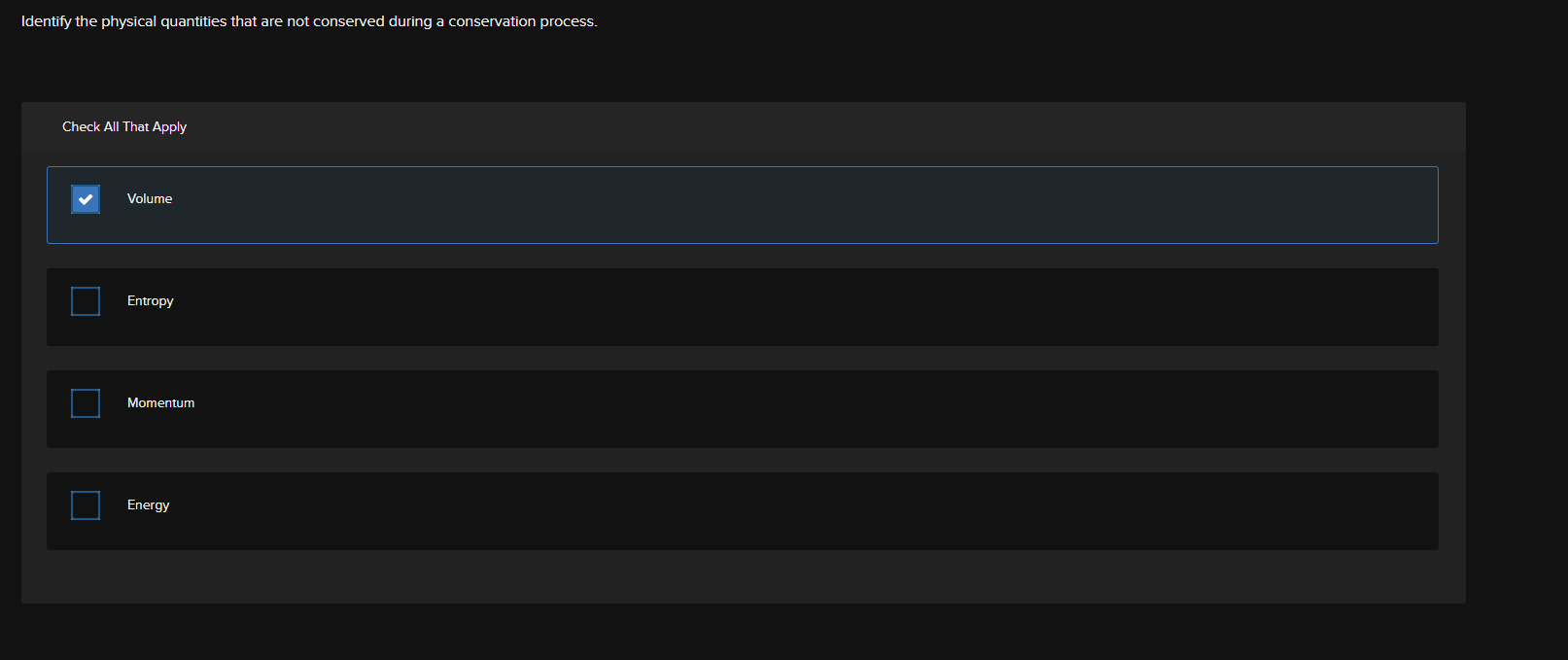The image depicts a structured quiz interface with a focus on identifying non-conserved physical quantities during a conservation process. The top portion features a black rectangle on the left, containing the instructional text in white: "Identify the physical quantities that are not conserved during a conservation process." Below this, there's a dark gray rectangle with smaller integrated rectangles. On the left side of this gray rectangle, in white capital letters, are the words "CHECK," "OR," "THAT," and "APPLY." 

The quiz includes four checkboxes. 

1. The first checkbox is blue with a white checkmark, labeled "VOLUN," highlighted in blue with a blue border shaping a rectangle around it.
2. Adjacent to the first checkbox, three smaller black rectangles are present with corresponding checkboxes. These checkboxes have a black interior and a blue outline. The label next to the first checkbox reads "ENTROPY," the second reads "MOMENTUM," and the third reads "ENERGY," all capitalized.

This detailed and organized layout effectively guides the user through identifying and selecting the appropriate physical quantities in the quiz.